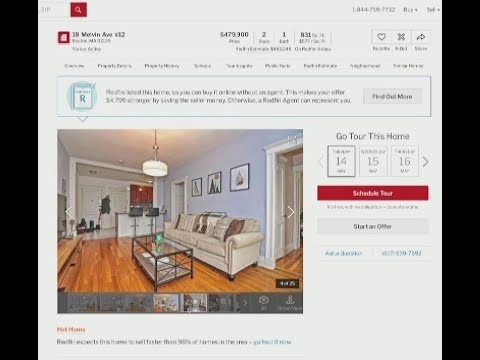This screenshot features a blurred image with largely unreadable text set against a black background on both the left and right sides. In the upper left corner, there is a red magnifying glass icon within a square, accompanied by a search bar labeled "ZIP." The upper right corner displays a phone number, likely 844-250-2232, in black text. Beneath a light gray line, an address appears, possibly "28 or 2B Melvin Ave, Unit 12," alongside a price of $479,900.

In the upper right corner, there are three interactive icons: a heart for liking, an "X" for closing, and an arrow pointing right. 

The lower center of the image showcases a color photograph of a living room. The room features a light blue wall, a cream-colored sofa positioned against it, and a glass coffee table in front of the sofa. The floor is wooden, and on the right side, there's an open doorway or hallway framed with white wood molding.